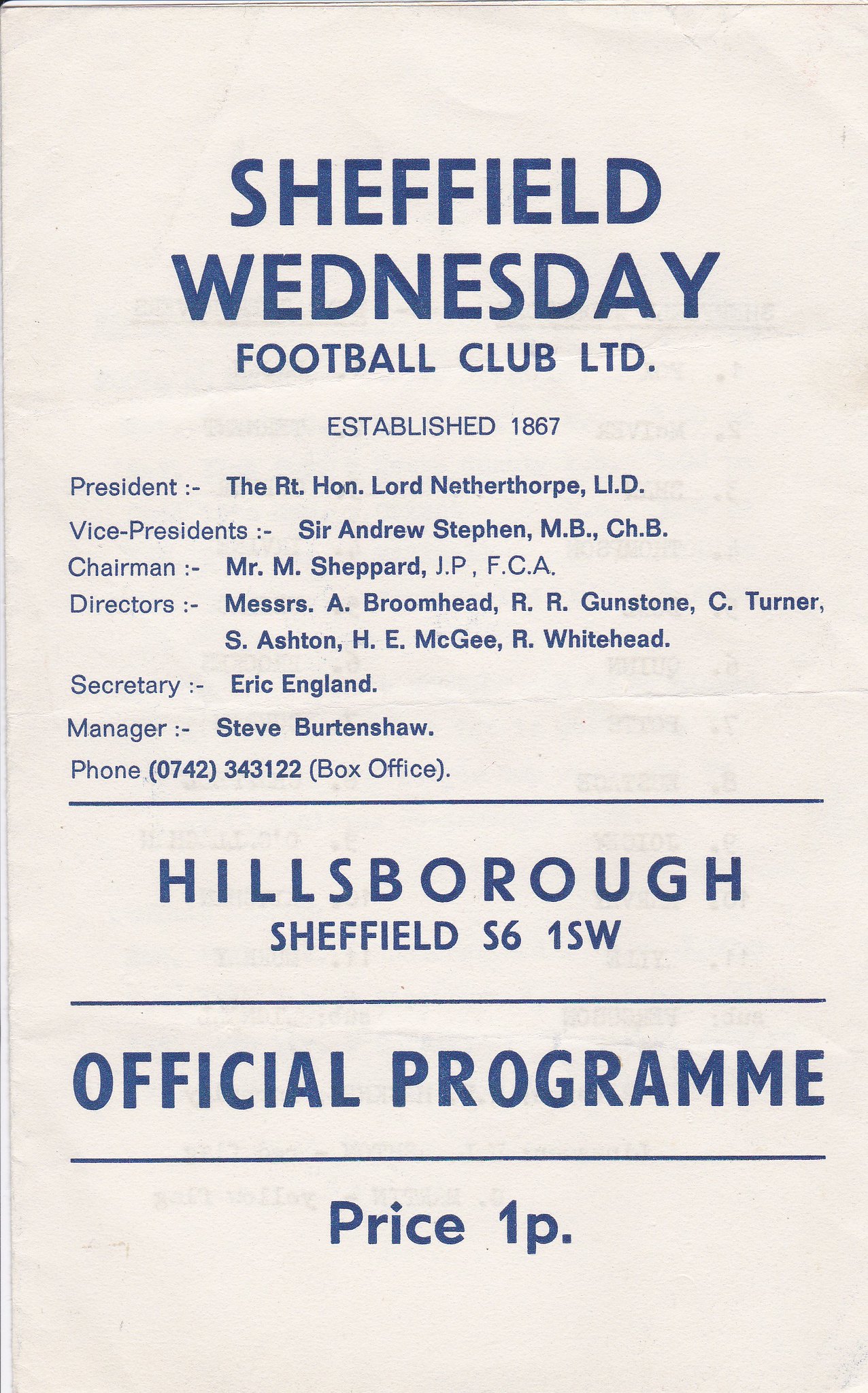This is the cover of an official program for Sheffield Wednesday Football Club. The vertical rectangular poster features dark blue lettering on a pinkish-white background. At the top, in large capital letters, it reads "Sheffield Wednesday Football Club, LTD" with "Established 1867" in smaller print beneath it. Below this, the poster lists the club's key personnel in a column: President, the Right Honorable Lord Netherthorpe, O.I.D.; Vice President, Sir Andrew Stephen, M.B.C.H.B.; Chairman, Mr. M. Sheppard, J.P.F.C.A.; Directors, Messrs. A. Broomhead, R.R. Gunstone, C. Turner, S. Ashton, H.E. McGee, R. Whitehead; Secretary, Eric England; and Manager, Steve Burtenshaw. 

Following this information, a phone number, "0-742-343-122," is provided alongside the note "Box Office." A horizontal blue line spans the poster below the column of names, with the text "HILLSBORO" in large blue letters underneath. The address "Sheffield, S6 1SW" follows, succeeded by another horizontal blue line. The phrases "OFFICIAL PROGRAM" and "Price: 1P." conclude the text, marking this document as the official program for a Sheffield Wednesday Football Club match.